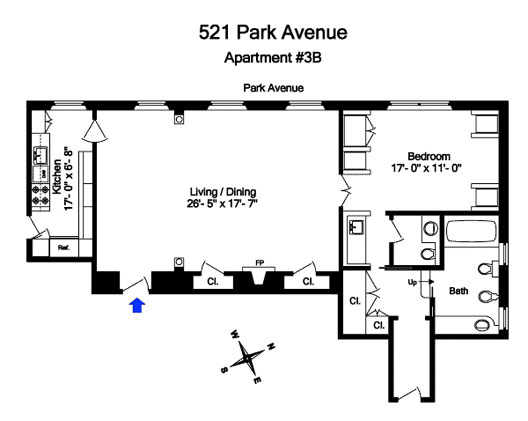"Detailed floor plan of 521 Park Avenue, Apartment 3B. The black-and-white schematic is marked at the top with the apartment number, where the number sign is referred to as a 'hashtag' in modern parlance. The layout includes:

- A galley kitchen on the left side, with specified dimensions.
- A large living/dining room measuring 26 feet 5 inches by 17 feet 7 inches, featuring a fireplace (labeled 'FP') flanked by two closets ('CL'), each with a door.
- A bright blue arrow highlights a section of the plan.
- In the bottom left corner, marked beneath the dining/living room area, is an exterior entry door swinging inward, presumably the main entrance from the hallway.
- A compass rose beneath this area indicates directions: West towards the top-left corner, North to the top-right, East to the bottom-right, and South to the bottom-left.
- Adjacent to the living/dining room is a spacious bedroom, sized 17 feet by 11 feet, illustrated with a bed and armchairs.
- Two bathrooms are shown: a full bathroom equipped with a tub, commode, and sink, and an additional powder room. Both bathrooms include closets.

The layout appears to be one-bedroom with additional amenities, although it features two bathrooms, raising some confusion regarding the overall arrangement."